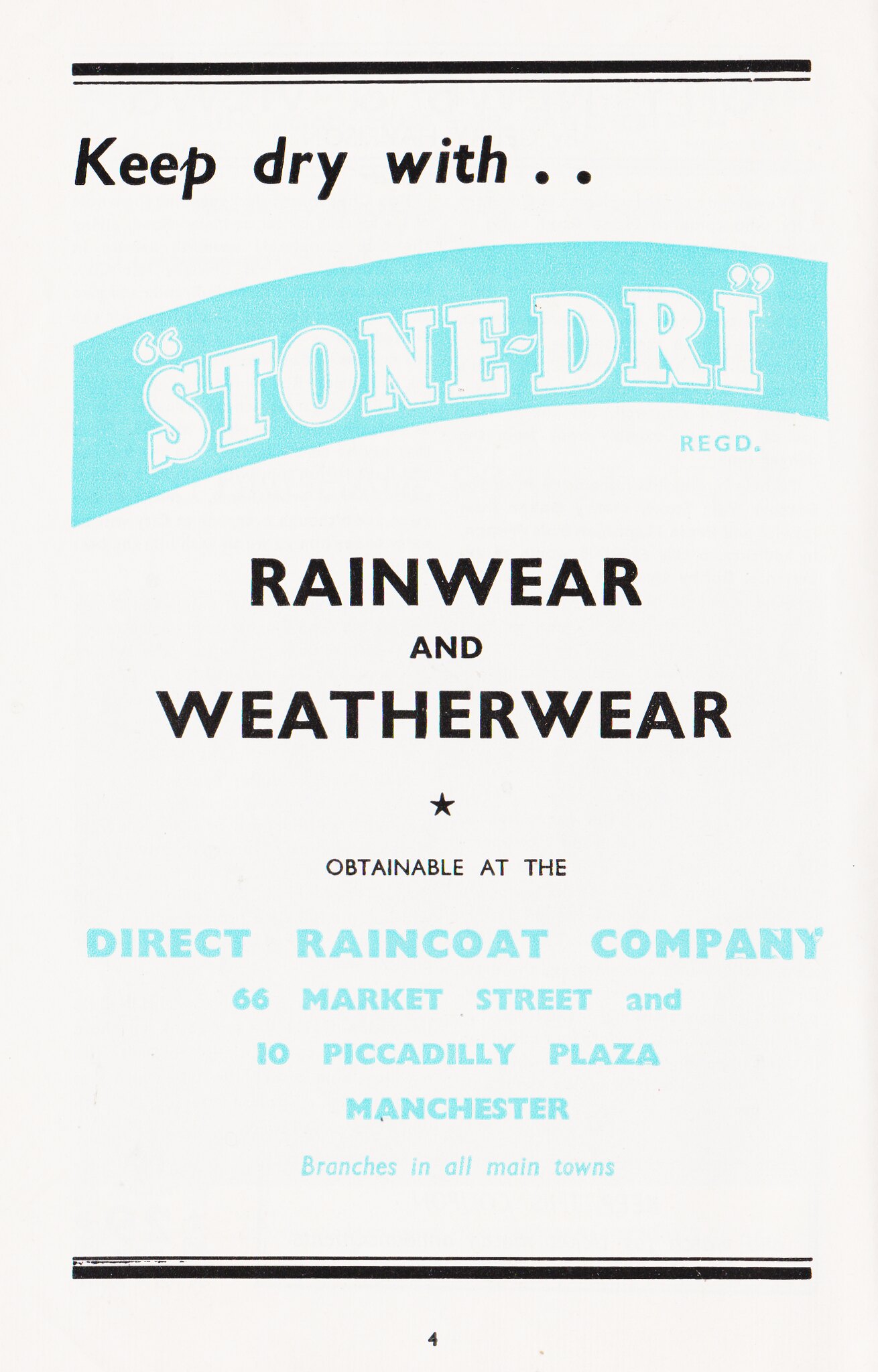The advertisement features a white background with a bold black line across the top. Below the line, in black font, it reads, "Keep dry with...". A turquoise, slightly diagonal banner follows, with the white text "STONE-DRI (Reg'd)". The text underneath in black font reads, "Rainwear and weather wear". There is a small black star below this line, followed by the text, "Obtainable at the Direct Raincoat Company," in turquoise font. The address "66 Market Street and 10 Piccadilly Plaza, Manchester. Branches in all main towns," is listed below. The bottom of the poster is bordered by a thin black line and a thicker black line, with the number 4 centered in black text.